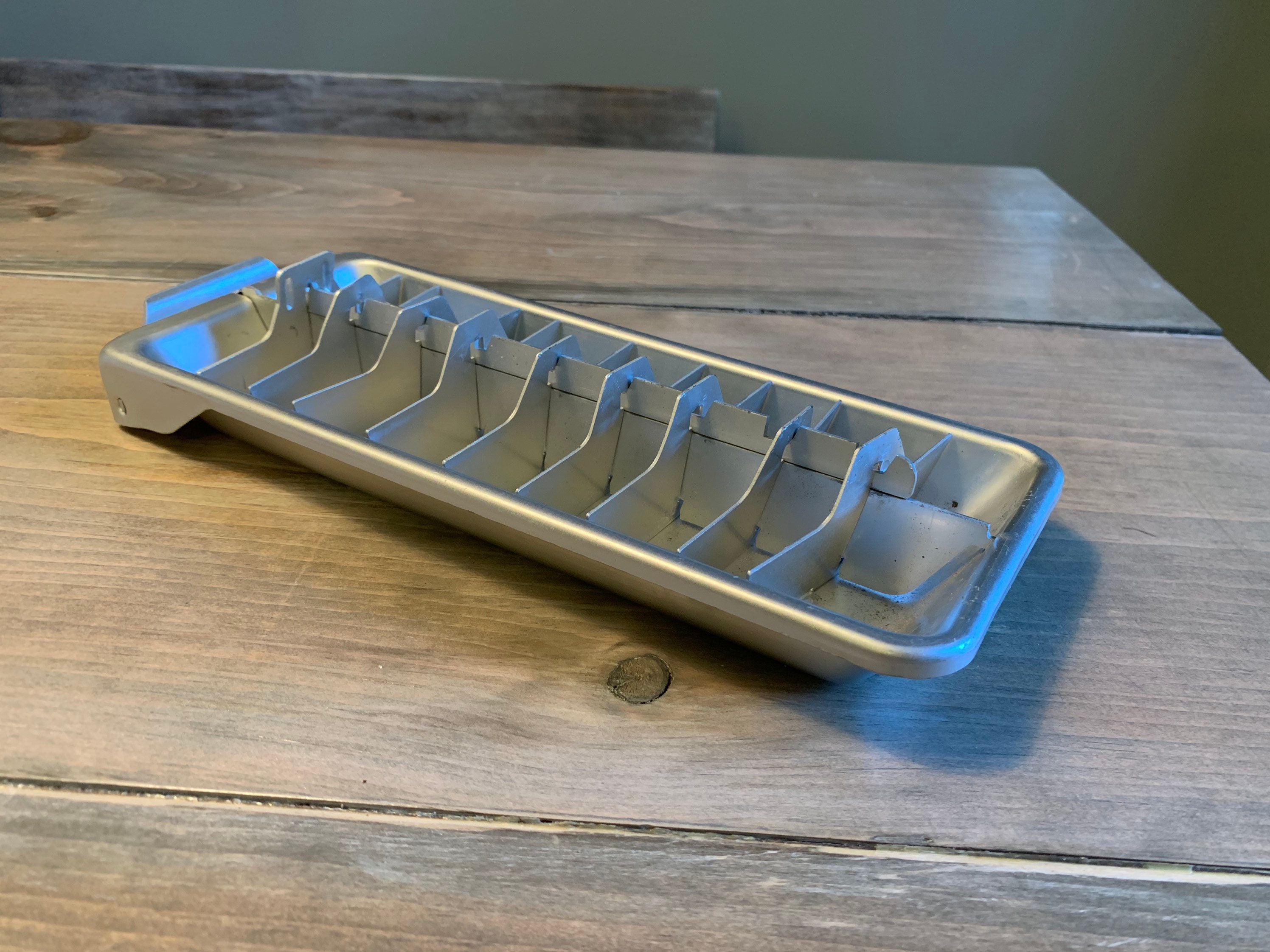The image depicts an old-fashioned, rectangular ice cube tray made of shiny, gray-colored metal, complete with silver dividers that form individual compartments approximately an inch apart. The tray, which appears new or well-maintained, features slightly rounded edges and a ridge-like handle at the back, positioned in the upper left corner of the picture. It rests on a dark brown wooden table, composed of three horizontal planks with noticeable knots, especially in the middle and upper left. Behind the table, there is a wooden chair or bench partially visible in the upper left corner. The background reveals a gray or army-green painted wall.